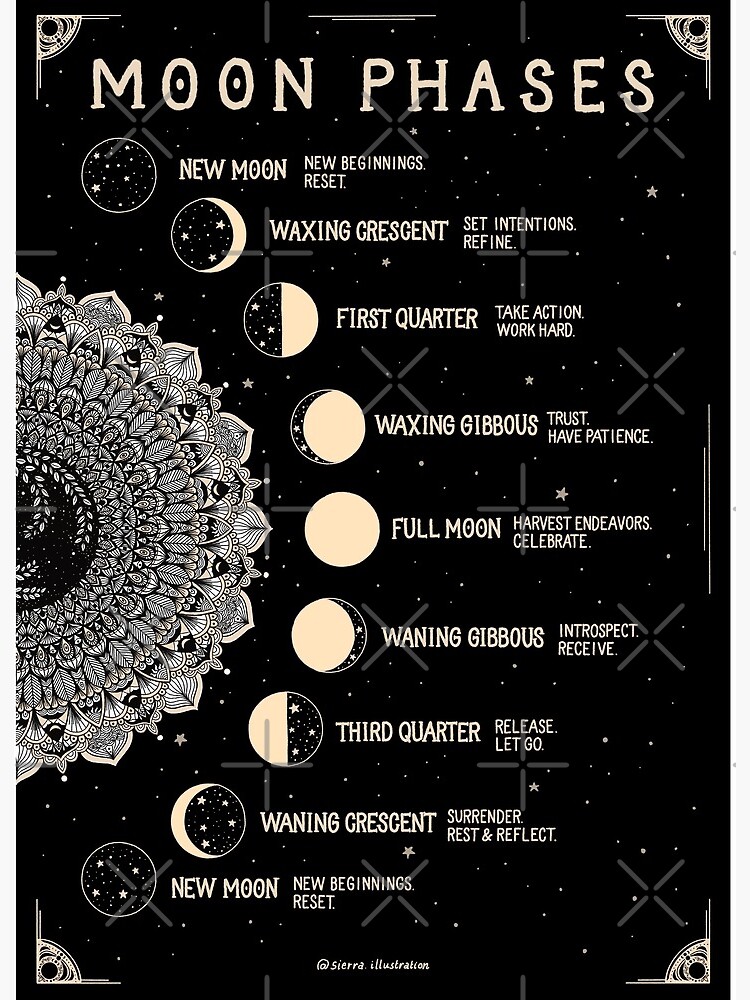This ornate and elegant black-and-white poster illustrates the phases of the moon. Titled "Moon Phases" at the top in a hand-script style font, this chart provides detailed descriptions for each lunar stage. The background is adorned with star patterns, while intricate filigree or scalloped designs decorate the corners. On the left side, there is a highly stylized half mandala, resembling multiple feathers or petals, which adds to the decorative nature of the poster.

The poster features the following lunar phases, each accompanied by a corresponding visual representation and text:
- **New Moon**: "New beginnings, reset."
- **Waxing Crescent**: "Set intentions, refine."
- **First Quarter**: "Take action, work hard."
- **Waxing Gibbous**: "Trust, have patience."
- **Full Moon**: "Harvest, endeavors, celebrate."
- **Waning Gibbous**: "Introspect, receive."
- **Third Quarter**: "Release, let go."
- **Waning Crescent**: "Surrender, rest, and reflect."
- **New Moon** (repeated): "New beginnings, reset."

The artwork is credited to Sierra Illustration, elegantly noted at the bottom of the poster. The layout and meticulous design elements suggest an astrological influence, making this poster not only informative but also visually captivating.